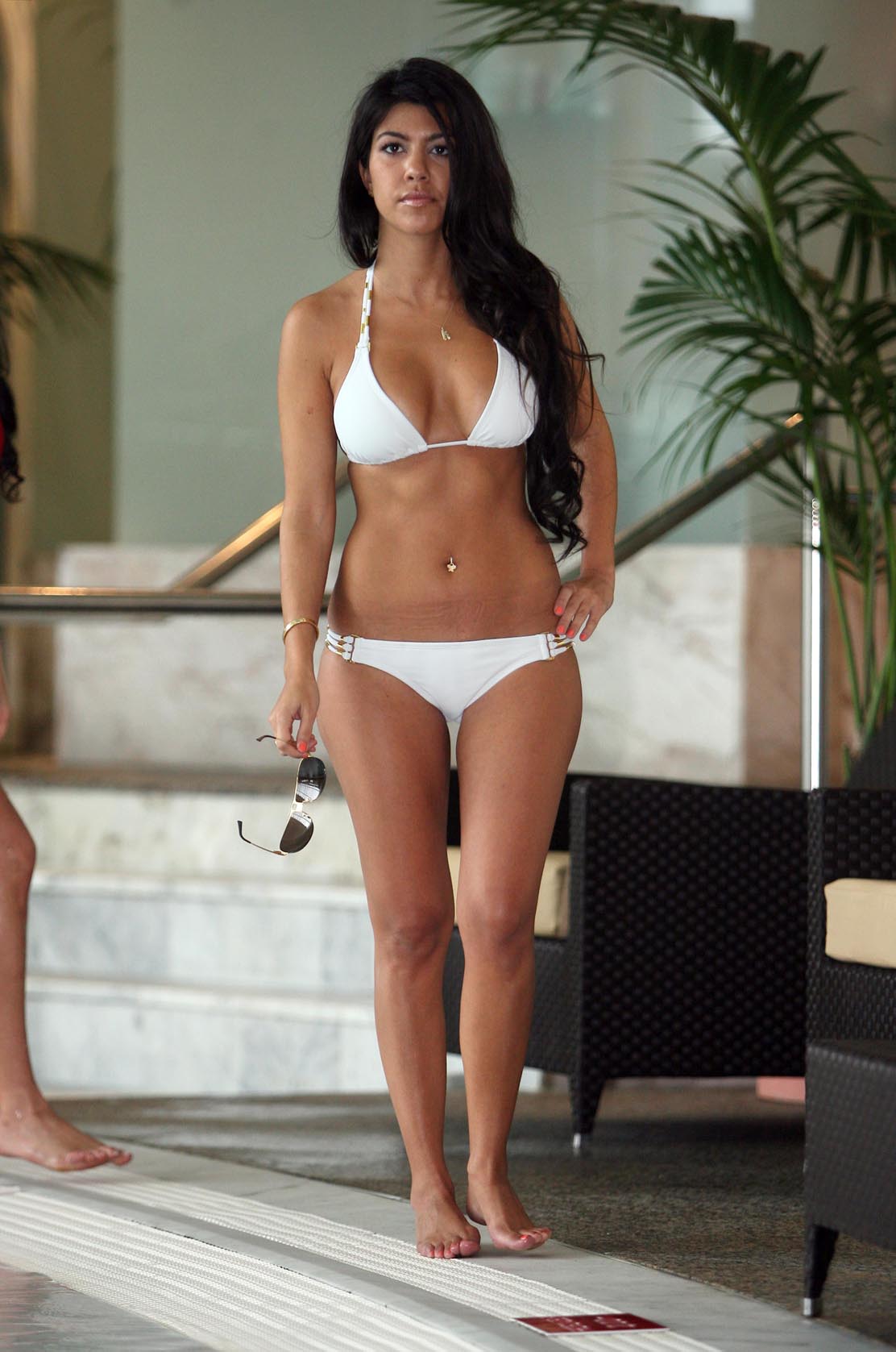The image showcases Kourtney Kardashian in a white bikini, resembling white underwear and a bra-like top, adorned with a gold, thin necklace and a navel piercing. Her long, flowing black hair cascades down toward her stomach, while she holds sunglasses and places her left hand on her hip. She is barefoot on a grey carpet, presumably near a pool area, possibly at a resort or her home. The scene includes black chairs with tan cushions, a fake palm tree, and a glass railing with marble steps in the background. Also visible is a foot beside Kourtney, hinting at the presence of another person, potentially another of her sisters.